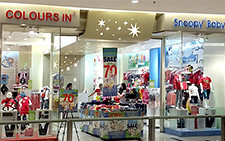The image depicts a brightly lit shopping mall scene, focusing on a children's store. Above the glass windows, there's a star motif. The upper left-hand corner displays a sign that reads "Colors Inn" in red text, and on the right side, another sign reads "Snoopy Bobby." In between, there are multiple signs indicating a sale, with one prominently stating "70% off." Another sign with the same message is placed on an easel to the left of the main sale sign. The store interior features colorful clothing displayed on mannequins dressed in white jeans and t-shirts, as well as a large bin in the middle of the store filled with colorful items. The background is predominantly beige, and the store is viewed through large glass windows.